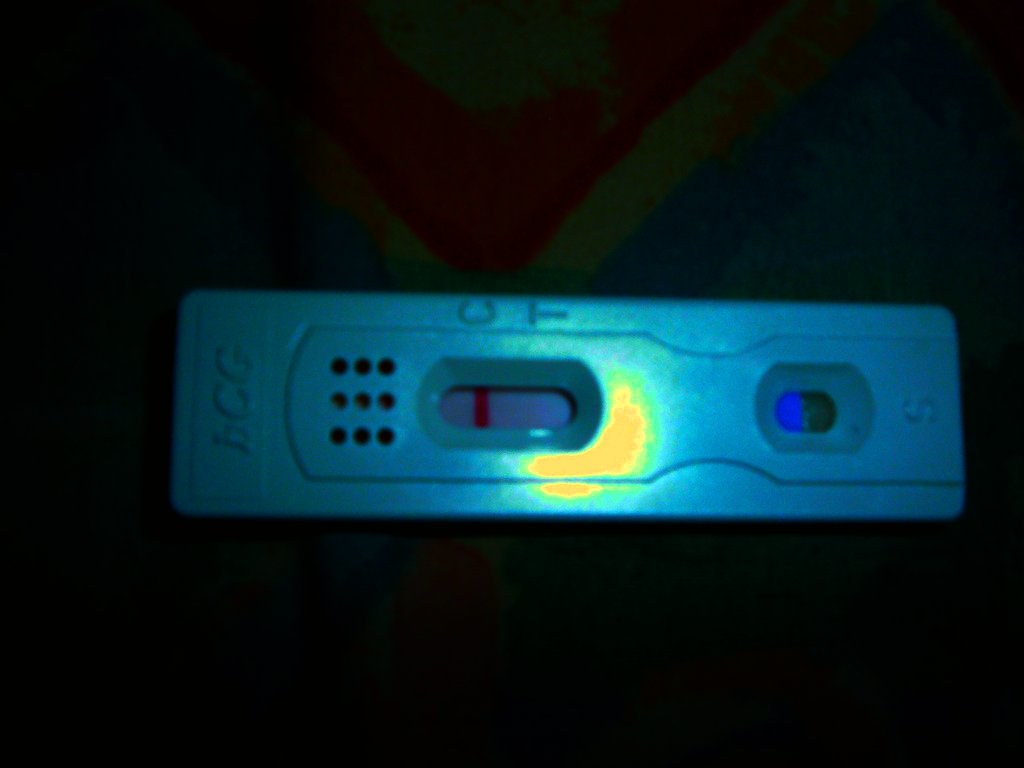This photograph features an instrument positioned against a completely black background. The instrument is rectangular, occupying approximately one-third of the total space of the image. Vertically centered, it is slightly off-center to the right of the horizontal axis of the black square. 

The instrument is a striking blue, likely made of metal given its reflective surface, which catches the light in places. Its design is reminiscent of a yellow banana with a subtle green hue outlining its shape. On the right side of the device, there's a small viewing window that is a light blue shade, which darkens to a deeper blue when exposed to liquid. This suggests it functions similarly to a pregnancy test or a COVID-19 test, where liquid moves across a test strip to show results.

In the middle of the instrument lies a larger, oval-shaped window displaying one red line, potentially indicating a test result, be it positive or negative. To the left of this window, there are three rows of three black dots, possibly sensors or indicators. 

The top of the device is embossed with the initials 'B', 'C', and 'G', hinting at a connection to the BCG (Bacillus Calmette-Guérin) vaccine or another related test.

Overall, this detailed medical instrument stands out vividly against the stark black background, showcasing its intricate design and functional elements clearly.